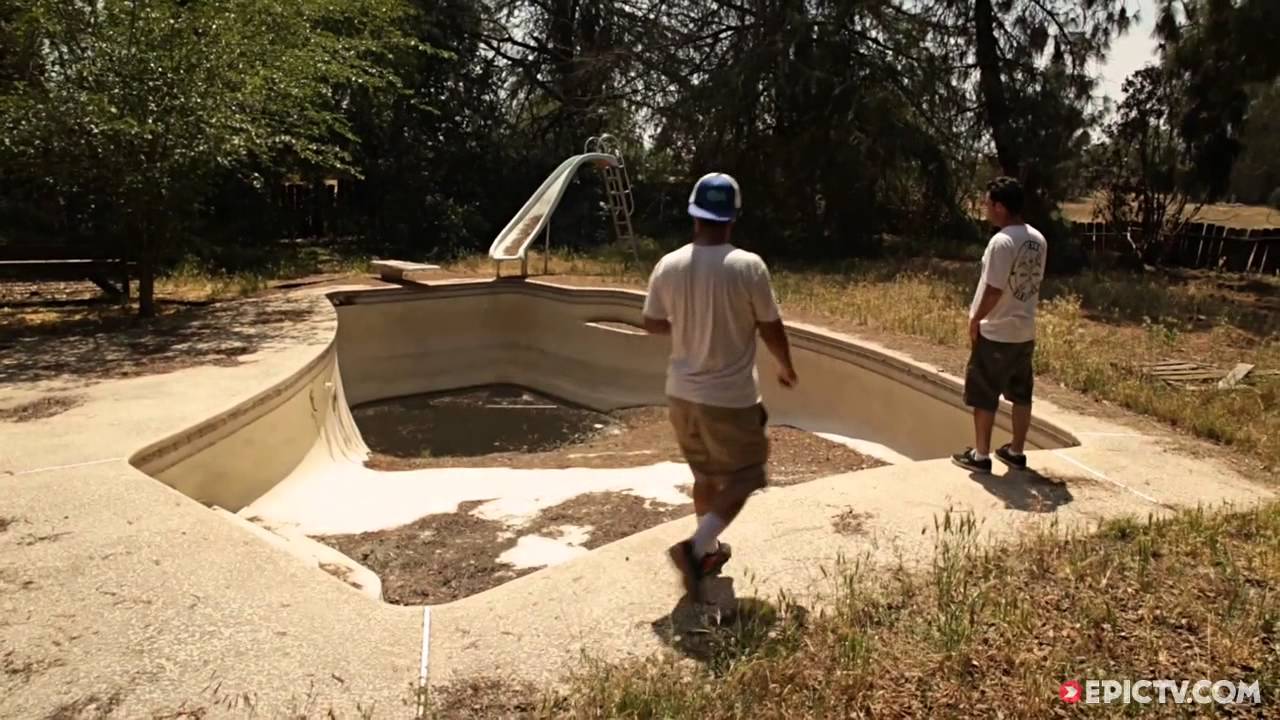Two men stand in an overgrown backyard, examining a large, empty in-ground pool that looks neglected and has not been used for some time. Both are dressed casually in T-shirts, shorts, and sneakers; one wears a backwards hat and the other black Vans. The pool itself is filled with leaves, debris, and has patches of standing water at the bottom, with dirt collecting in various spots. This non-traditional shaped pool, outlined in light brown or beige concrete, features both a slide leading towards the deep end and a diving board. Surrounding the pool, the yard is unkempt, with tall grass and weeds overtaking the area. In the background, there are scattered trees and a single-story wooden building or shack. A park bench is also visible to the left, further accentuating the scene's abandonment and disrepair.